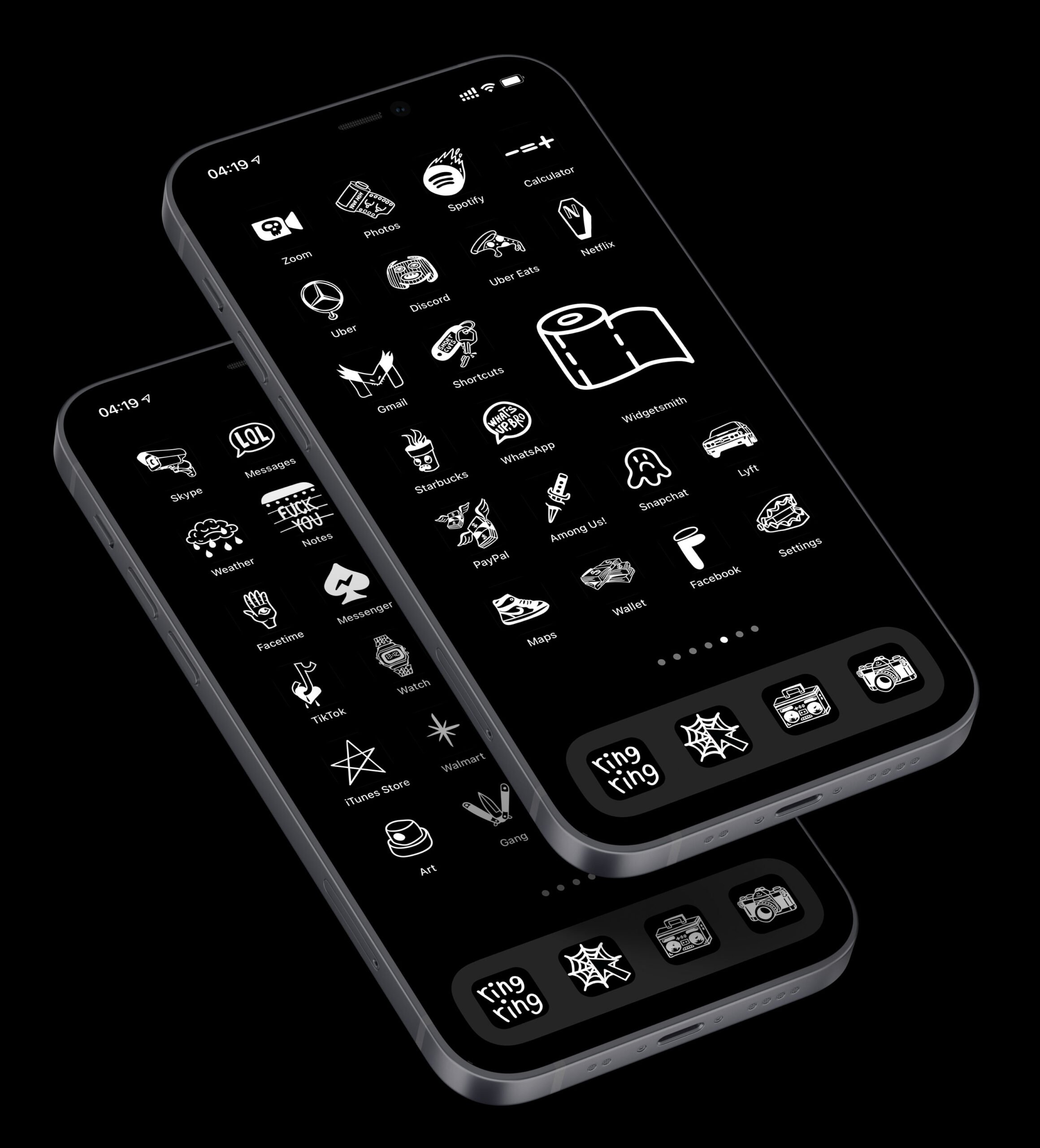The image displays two black smartphones against a black background, positioned one atop the other with the top phone elevated diagonally. Both screens share a plain black home screen background and showcase multiple app icons in white. On each screen, the current time, network status, and battery life are visible at the top. The screens feature apps such as Zoom, Discord, Uber, WhatsApp, Snapchat, Photos, Spotify, Calculator, Uber Eats, Netflix, Gmail, Shortcuts, Starbucks, WidgetSmith, PayPal, Among Us, Lyft, Maps, Wallet, Facebook, and Settings. At the bottom, three navigation apps are visible in a lighter gray area. Multiple dots indicate several pages of apps. The phone's physical characteristics are further detailed by a visible USB port at the bottom and three buttons along the left side.